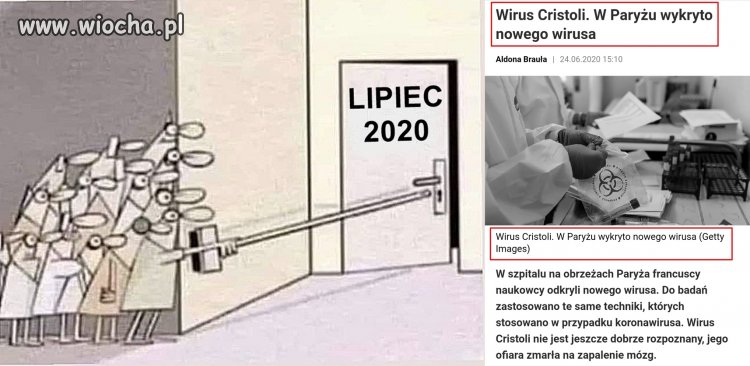The image is a detailed, cartoon-style illustration set up for circulation on social media. Dominating the left side of the image, which is primarily brown, tan, white, red, and black in color, is a black and white line art scene with a pink-colored floor. This scene features a group of digitally represented people, some in lab coats, huddled around a corner in a hallway. One person extends a broomstick towards a door labeled "Lipiec 2020," cautiously attempting to open it. On the right side, the image transitions into a real-life black and white photograph depicting a medical setting, where a doctor or surgeon is holding a biohazard bag. At the top left, the website "www.wiocha.pl" is clearly visible, indicating a Polish origin. The remainder of the text on the screen is in Polish and unreadable, suggesting the image could be an ad or feature for a Polish newspaper or publication.